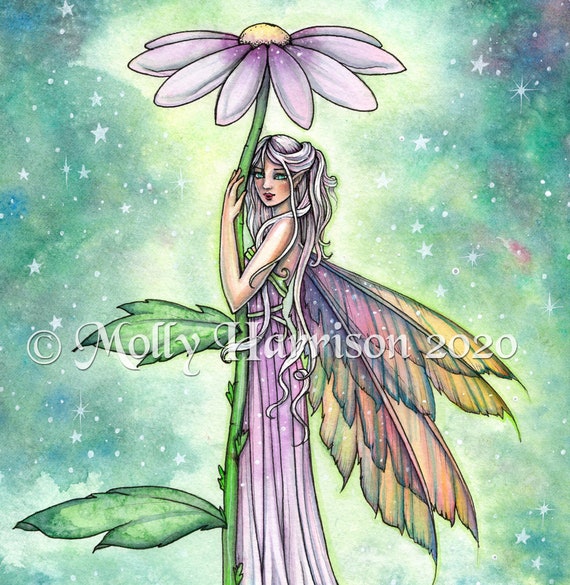The image is a detailed pencil drawing of a fairy, occupying the central position within a square frame. Across the center, there is a semi-transparent white watermark that reads "copyright Molly Harrison 2020." The fairy is embracing a green flower stem, which features two pointed green leaves and is topped with a purple flower boasting delicately detailed petals and a yellow center. The fairy is elegantly dressed in a sleeveless, long purple gown that extends to the bottom of the image. Her cascading white hair flows down past her waist. She possesses a set of four semi-transparent wings in pastel shades of green. The background depicts a sky in varied hues of light blue, teal, and green, adorned with scattered white stars, resembling a cosmic scene. The fairy's gaze is directed slightly to the left.